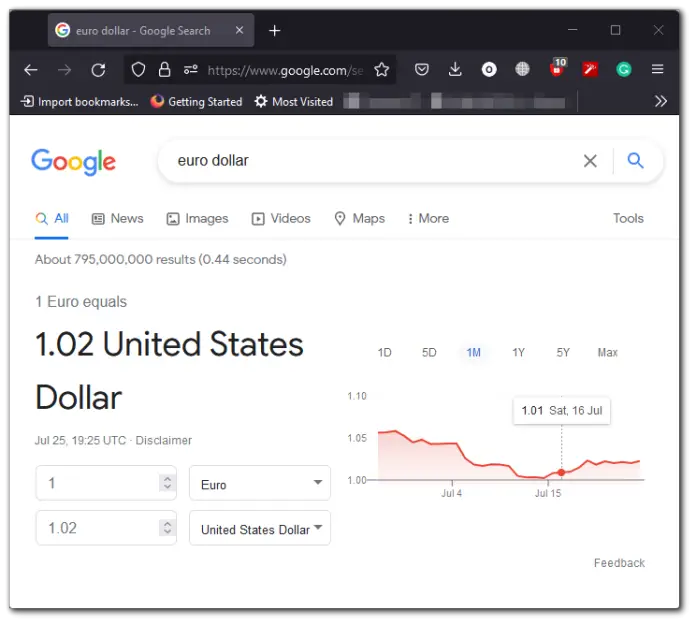The image captures the results of a Google search for "Eurodollar." At the top, within a black header bar, the text "Eurodollar - Google Search" is prominently displayed, confirming the search engine in use. Below this header, the address bar reads "google.com," accompanied by various navigation icons including a back button, a refresh button, a download icon, and another refresh button.

The main content area features the recognizable Google logo on the top left, adjacent to a search bar containing the term "Eurodollar." Directly beneath the search bar are the typical Google navigation options: All, News, Images, Videos, Maps, and More.

The search results highlight the current exchange rate between the United States Dollar (USD) and the Euro (EUR), indicating that 1 Euro is equivalent to 1.02 USD. To the right of this information, a graph illustrates the fluctuation in the dollar’s value over time. Beneath the exchange rate, dropdown boxes allow users to convert between currencies, showing "1 Euro" and "1.02 United States Dollar."